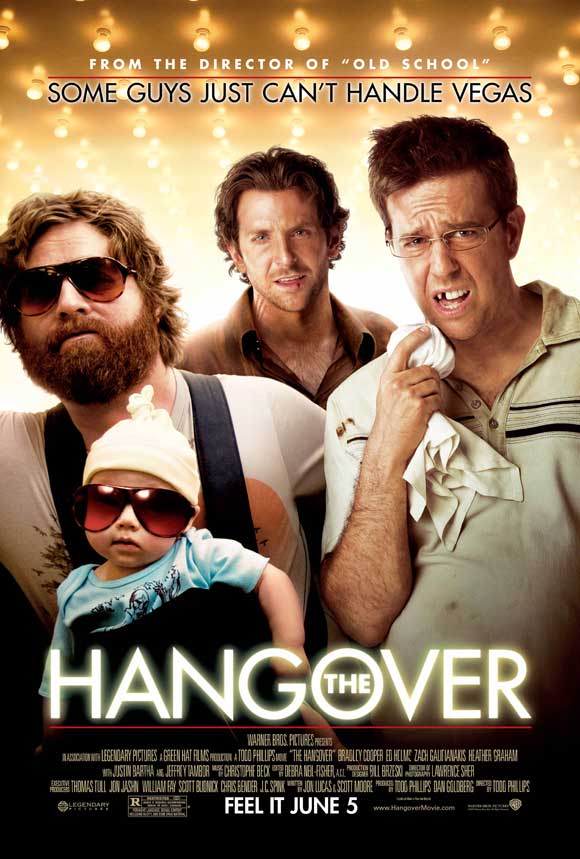This detailed movie poster for "The Hangover" prominently features a trio of disheveled men against a backdrop of lit bulbs, suggesting the bright lights of Las Vegas. At the top, the text reads, "From the director of Old School," followed by a tagline, "Some guys just can't handle Vegas." The central image showcases the film's stars: on the left stands a bearded man with scruffy hair and sunglasses, identified as Zach Galifianakis, who has a baby in a front-facing baby carrier. The baby, matching his caregiver's look, also sports sunglasses and a white beanie with a blue shirt. To their immediate right is Bradley Cooper, characterized by his brown hair and a brown shirt, bearing visible scratches on his neck and lip. On the far right is another man, noted for his missing tooth, glasses, and a blue-striped button-up shirt, holding a cloth to his mouth, implying a recent altercation. At the bottom, large text spells out "The Hangover," with "The" encased within the "O" of "Hangover." Below this, a red line underlines the credits listing the cast and crew, culminating in the release prompt, "Feel it, June 5th." This poster captures the chaotic allure of the film, hinting at the comedic misadventures that await.